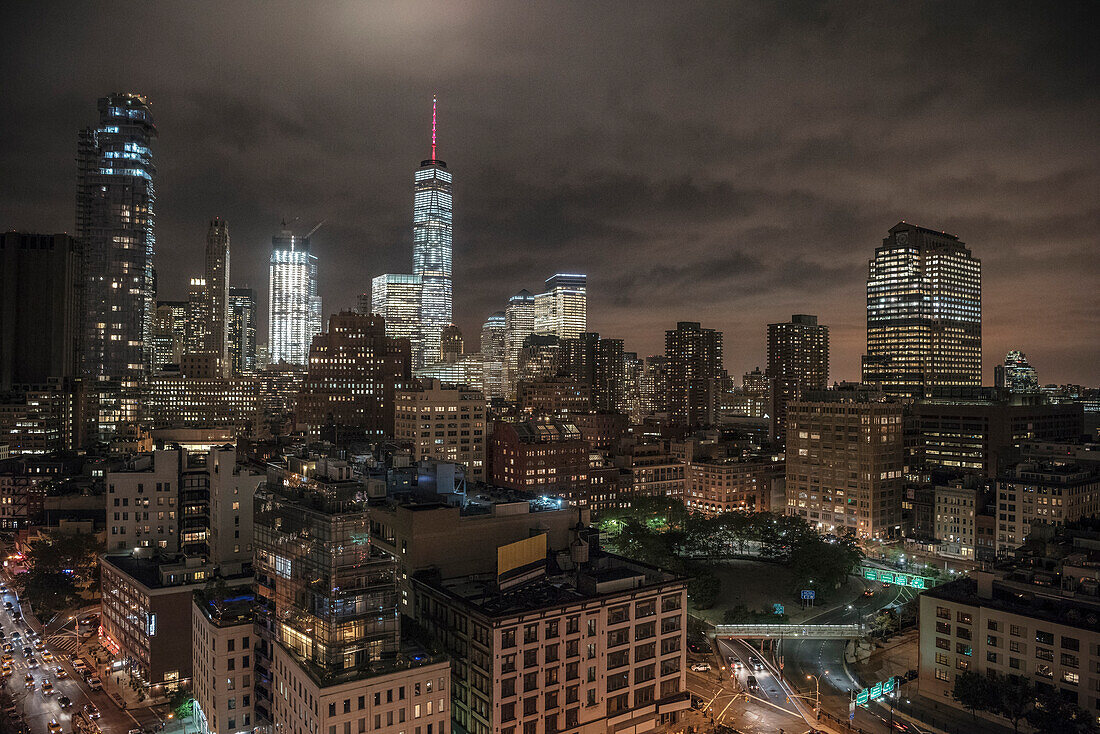This is a high-resolution, photorealistic aerial view of a sprawling metropolis at night, with an impending storm casting a dramatic ambiance. The dark, cloudy sky, tinged with a warm gray and hinting at red, suggests an approaching storm. There's a pronounced light source from above, potentially a helicopter illuminating the scene. Dominating the left side of the image is a cluster of towering skyscrapers, vividly lit, the most prominent of which features a striking pink spire at its peak. The surrounding buildings, though illuminated, are dwarfed in comparison and emit a subtler glow. A bustling freeway with numerous cars can be seen in the bottom left-hand corner, indicating heavy traffic, while the bottom right foreground reveals a dark park shrouded in shadows, making it difficult to discern specific details within. The cityscape, an intricate mix of varying building heights and extensive windows, displays a vibrant, active urban environment under the night sky.